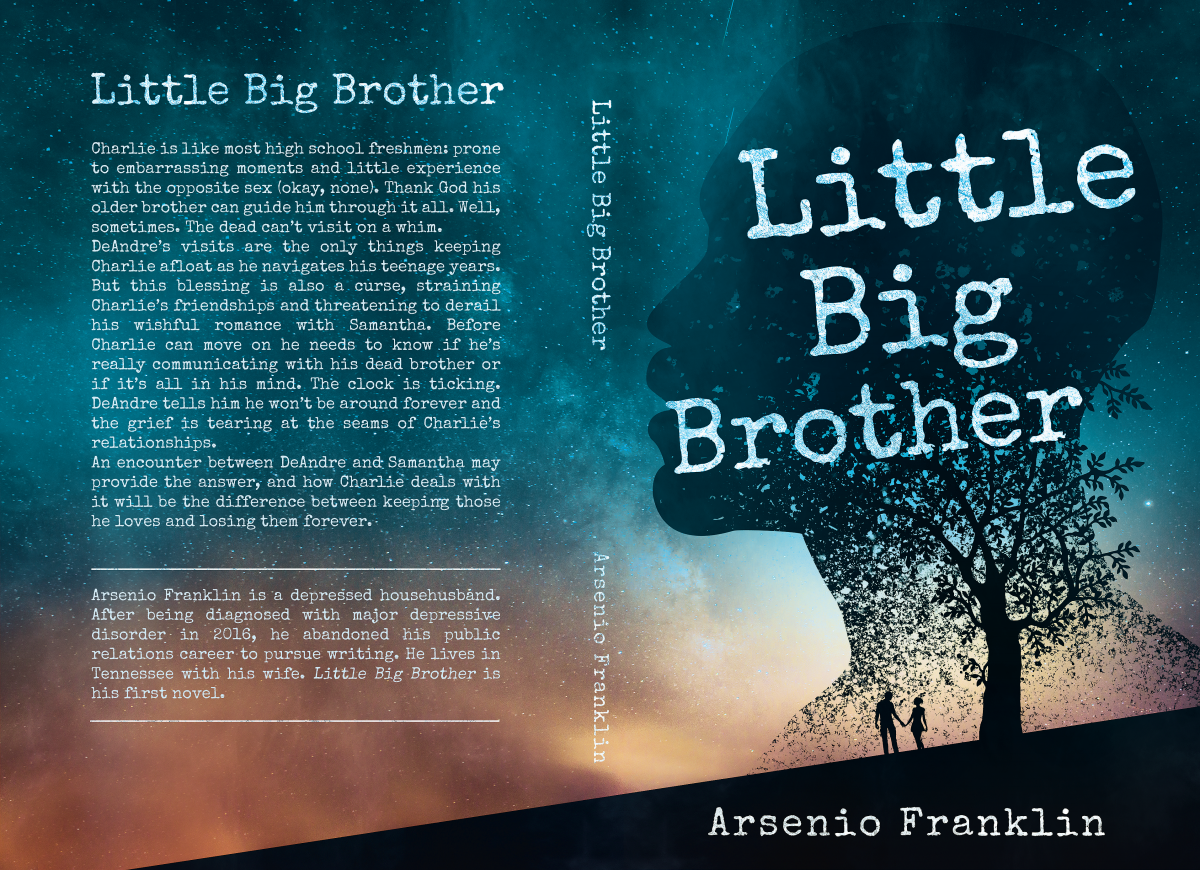The image depicts the front and back covers of the book "Little Big Brother" by Arsenio Franklin. The front cover is primarily blue, green, white, black, brown, and orange, and features a prominently large silhouette of a person's head at the top with a tree merging into the silhouette. Below, two people, a man and a woman, stand on the edge of a cliff, symbolizing the themes of the story. The back cover contains a summary of the plot where text highlights Charlie, a high school freshman experiencing awkward moments and lacking experience with the opposite sex. He is guided through these tumultuous teenage years by the ghost of his older brother, DeAndre. This supernatural guidance, however, also complicates his relationships, especially with a girl named Samantha. The story centers on whether Charlie is genuinely communicating with his deceased brother or if it’s a figment of his mind, a theme intertwined with navigating grief and adolescence. The back cover also provides information about the author, Arsenio Franklin, who shifted to writing after being diagnosed with major depressive disorder in 2016. The book appears as if displayed in an online marketplace, aiming to attract consumers with its captivating and emotional storyline.